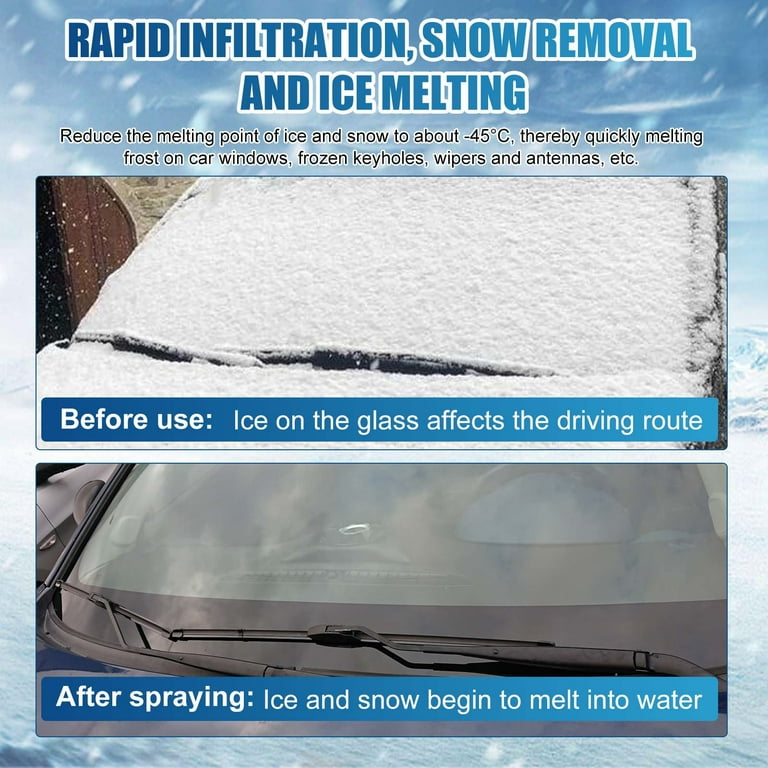This square-shaped advertisement vividly illustrates the effectiveness of "Rapid Infiltration Snow Removal and Ice Melting." The image background depicts a serene, icy, snowy day with blue skies and white, cloud-like snow, evoking a cold winter atmosphere. The centerpiece consists of two horizontally rectangular photographs: the top one shows a car's windshield entirely encrusted with thick snow, almost engulfing the wipers, while the bottom photo displays the same windshield, now almost clear and free of ice, suggesting the successful application of the product. 

In large, capitalized blue letters outlined in white, the caption at the top reads, "RAPID INFILTRATION, SNOW REMOVAL AND ICE MELTING." Below this, in black font also outlined in white, the text explains, "Reduce the melting point of ice and snow to about -45°C, thereby quickly melting frost on car windows, frozen keyholes, wipers, and antennas." 

A blue text box labels the top photo with "BEFORE USE: Ice on the glass affects the driving route," highlighting the dangerous obstruction. Correspondingly, the bottom photo is labeled "AFTER: Spring ice and snow begin to melt into water," indicating the efficacy of the product. The entire composition successfully showcases the dramatic before-and-after transformation, emphasizing the rapid melting action in a visually compelling snowy landscape.